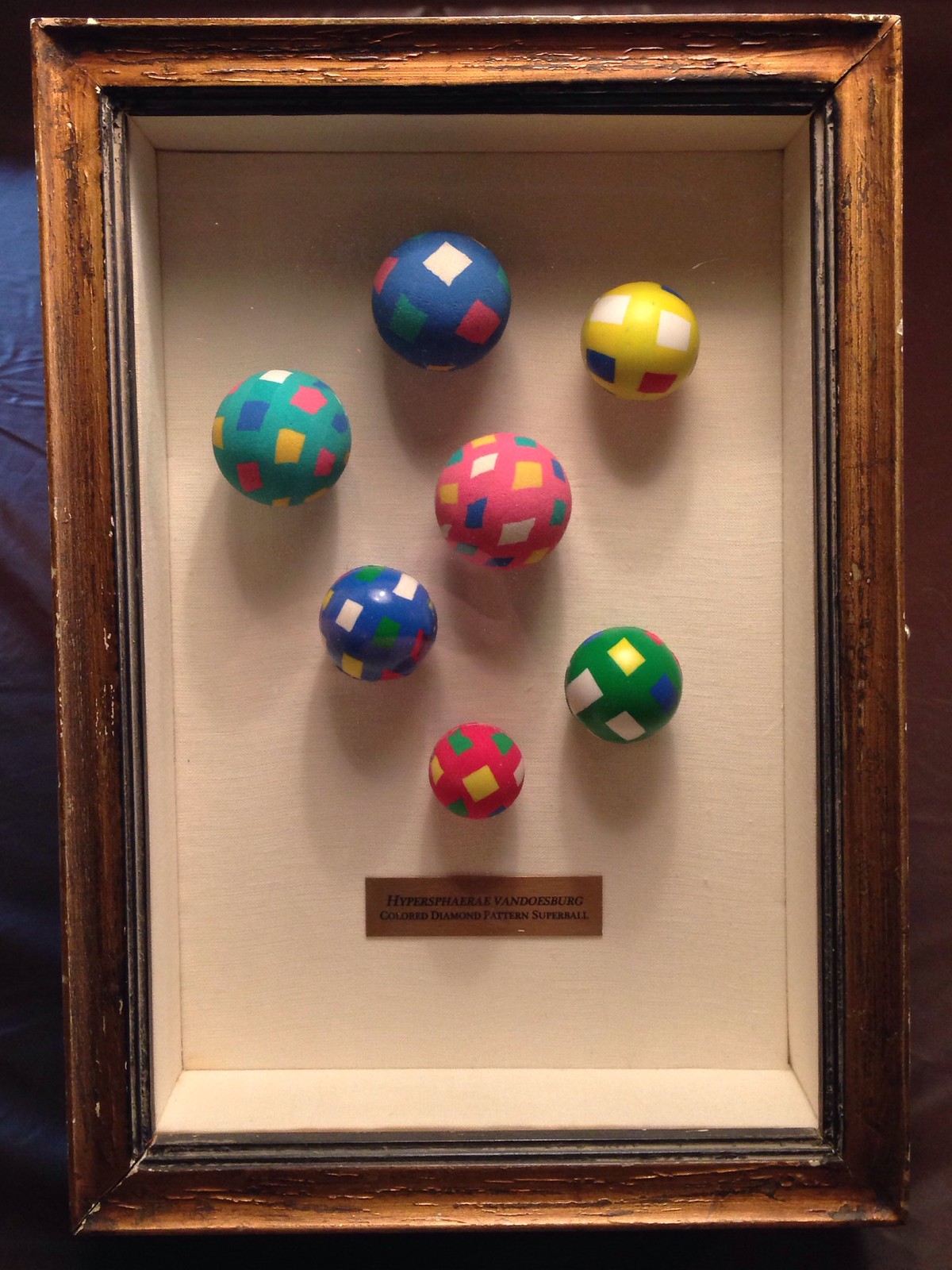This photograph captures a three-dimensional display, likely an art or museum piece, featuring a collection of colorful Super Balls. Encased in a worn, medium-toned wooden shadowbox frame with a blush liner, the display cradles seven vibrantly colored Super Balls of varying sizes. These balls are meticulously arranged in three rows: two on the top row, three in the middle, and two on the bottom. The balls, ranging from large to small, exhibit a spectrum of colors including teal, blue, pink, red, green, and yellow, each adorned with an intricate pattern of colored squares and diamonds. The backdrop of the display is a tan color, adding a neutral canvas to highlight the vibrant balls. A gold plaque with black lettering at the bottom of the display reads "Colored Diamond Pattern Super Ball" and bears the title "Hypersphere Vandesberg", hinting at the possible name of the artwork or collection. The overall condition of the display case suggests age and history, with the wooden frame showing signs of wear, adding a vintage charm to the piece.